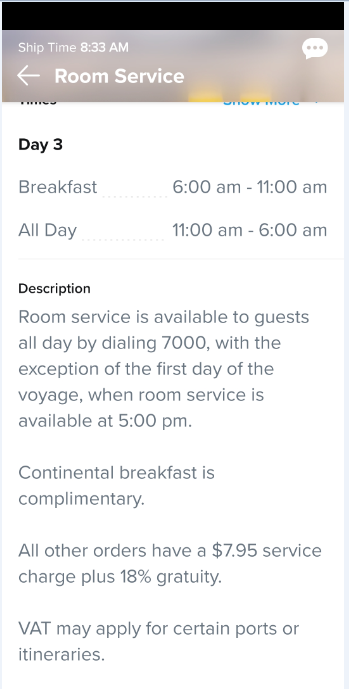This image is a screenshot of a cell phone displaying detailed room service information. Across the top, there's a thin black bar. Directly below it is a grey background bar featuring white text. At the top, it reads, "Ship Time, 8.33 AM." Beneath that, there's a left-pointing arrow followed by the text "Room Service," and on the right-hand side, a speech bubble with three dots in it.

The rest of the screen displays a white background with black and grey text. At the top, it reads, "Day Three," followed by specific meal times: "Breakfast, 6 AM to 11 AM" and "All Day, 11 AM to 6 AM." Below this, a description in black text provides further details: "Room service is available to guests all day by dialing 7000, with the exception of the first day of the voyage when room service is available at 5 PM. Continental breakfast is complimentary. All other orders have a $7.95 service charge plus 18% gratuity. VAT may apply for certain ports or itineraries."

Additionally, the image features vertical lines in very light grey on either side, indicating that there are elements cropped out of this particular screenshot. The layout and information are clearly intended to provide ship passengers with comprehensive details about room service availability and charges.